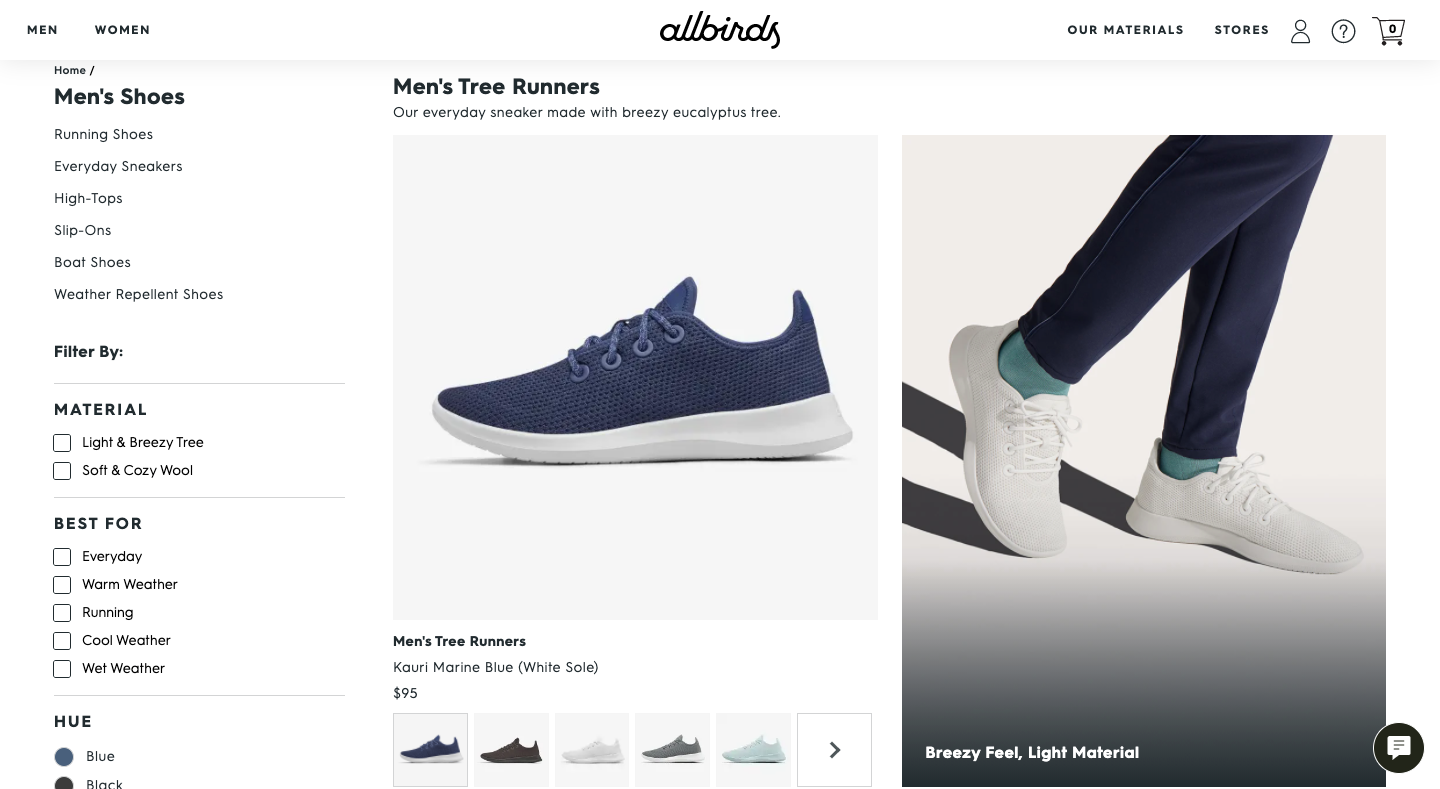The image is a screenshot from an online shopping website. At the top in a white space, bold black capital letters indicate categories such as "MEN" and "WOMEN." Centered on the page, the brand name "allbirds" appears in lowercase script. To the right, additional navigation options in capital letters include "OUR MATERIALS" and "STORES." Adjacent icons display a shopping cart, a help symbol represented by a circle with a question mark, and a profile icon depicting a head and shoulders.

Below, on a light gray background, text options appear such as "HOME," "MEN'S SHOES," "TYPE OF SHOES," and filters like "FILTER BY MATERIAL," and "BEST FOR." Categories include "HUE," allowing color selection. Prominently in the center, the product section labels "MEN'S RUNNING" and "MEN'S TREE RUNNERS." Accompanying graphics showcase a single blue shoe with a white sole, accompanied by its price and five alternative color options.

Adjacent in a separate panel, another graphic features a gradient background transitioning from dark to light gray. It displays a person shown from the knees down, dressed in blue loose-fitting leggings, teal socks, and white shoes.